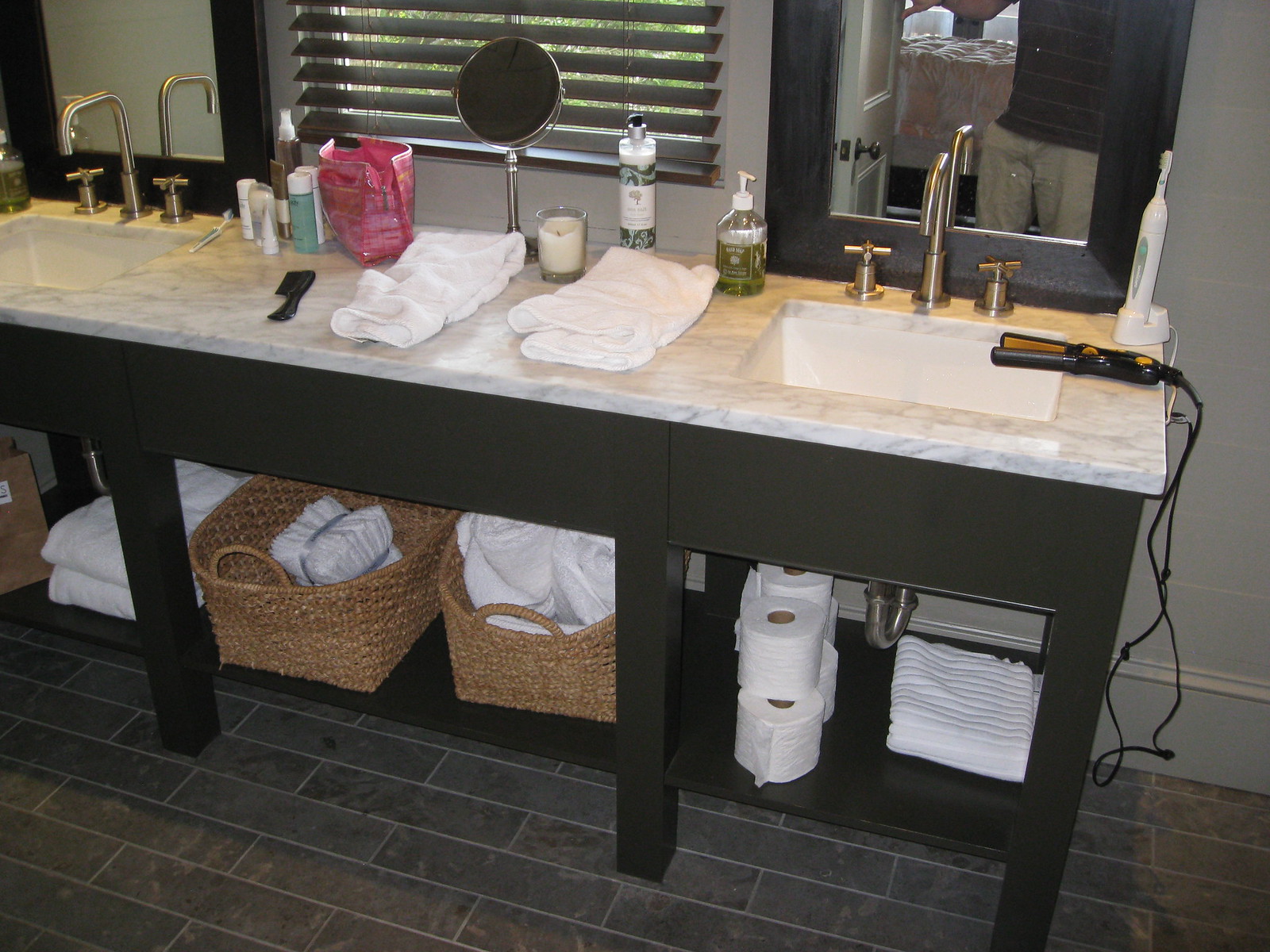This image captures a spacious hotel bathroom featuring dual identical sinks. Between the sinks, neatly arranged towels are visible. On the right side of the countertop, a plugged-in hair straightener is poised for use. A comb is placed on the left side of the countertop. Below the sinks, a wicker basket overflowing with additional towels is visible. Various soap products are arrayed on the countertop, adding convenience and luxury to the setting. The overall atmosphere combines practicality with an inviting aesthetic.